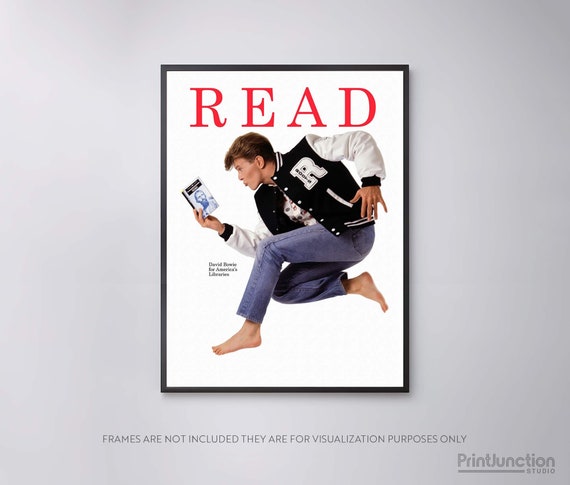This image portrays a vintage poster in a thin black frame, featuring a young man, likely from the late teenage years or early twenties, with brown hair. He is dressed in a black Letterman jacket with white sleeves, displaying the letter "R" prominently, paired with blue jeans and bare feet. The young man is captured in mid-movement, appearing to dance while holding a blue-covered book in his right hand. The book's cover depicts a person with a beard, possibly referencing Julius Caesar. Above the young man, the word "READ" is prominently displayed in bold letters. Below his crouched stance, legible text indicates "David Bowie for America's libraries." The background of the image is white, and additional text in the bottom right corner reads "Print Junction Studio" in gray. A note clarifying that "frames are not included" and are "for visualization purposes only" is visible outside the main image area. Overall, the poster combines elements of 80s nostalgia with an educational message.